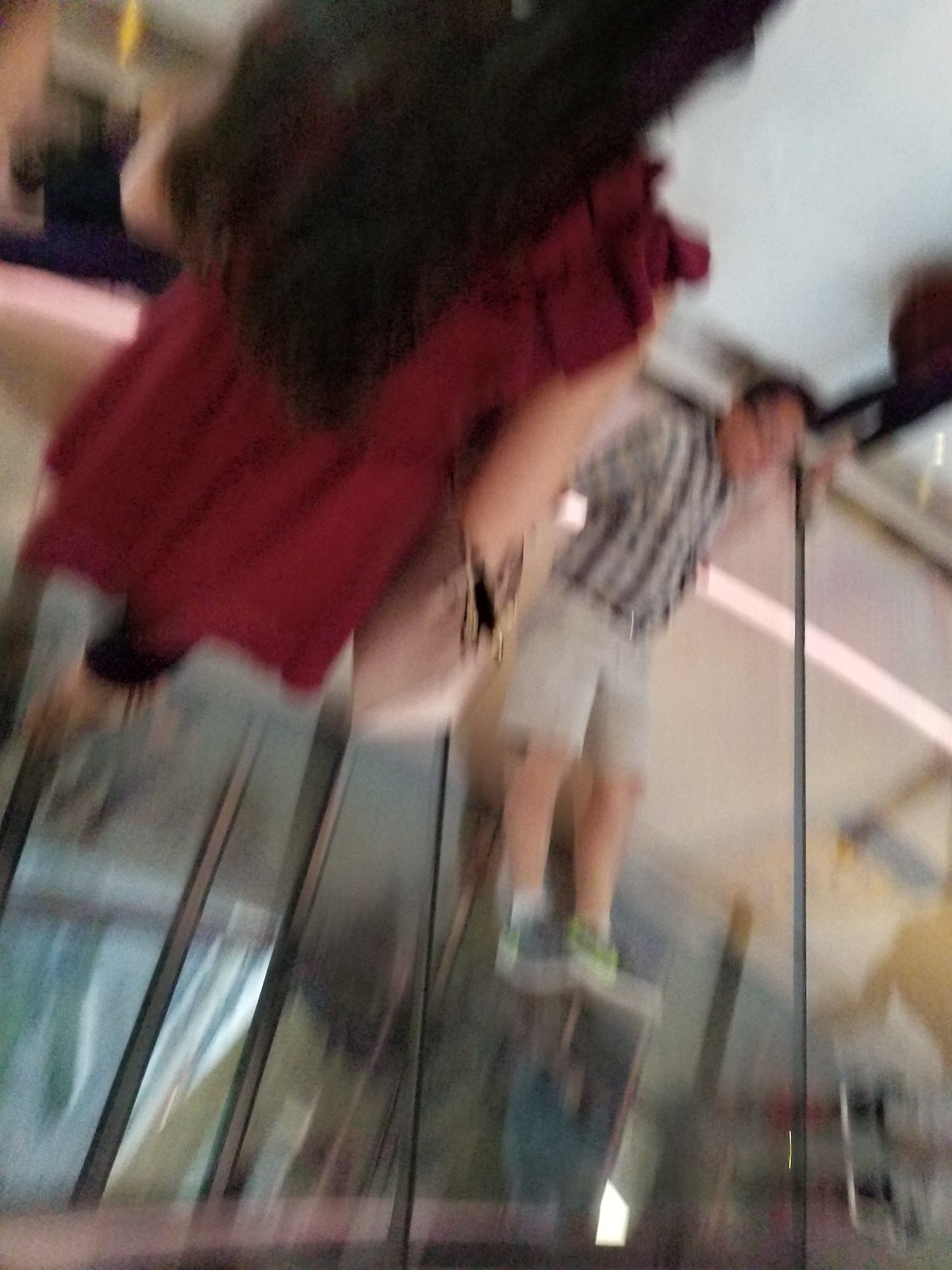The photo captures two individuals, possibly of Caucasian or Asian descent, in a slightly ambiguous setting due to its blurriness. The man is seated against a beige-colored wall, dressed in a plaid shirt, khaki pants, and tennis shoes, with a pair of glasses perched on his nose. Directly beneath him, there is a clear glass surface, adding an intriguing element to the scene. A woman stands beside him, wearing a red burgundy dress paired with dark tights, and carrying a bag. She has long, brown hair cascading down her shoulders. The duo appears to be situated on a see-through walkway, which might explain why they appear apprehensive or uneasy in the photo.